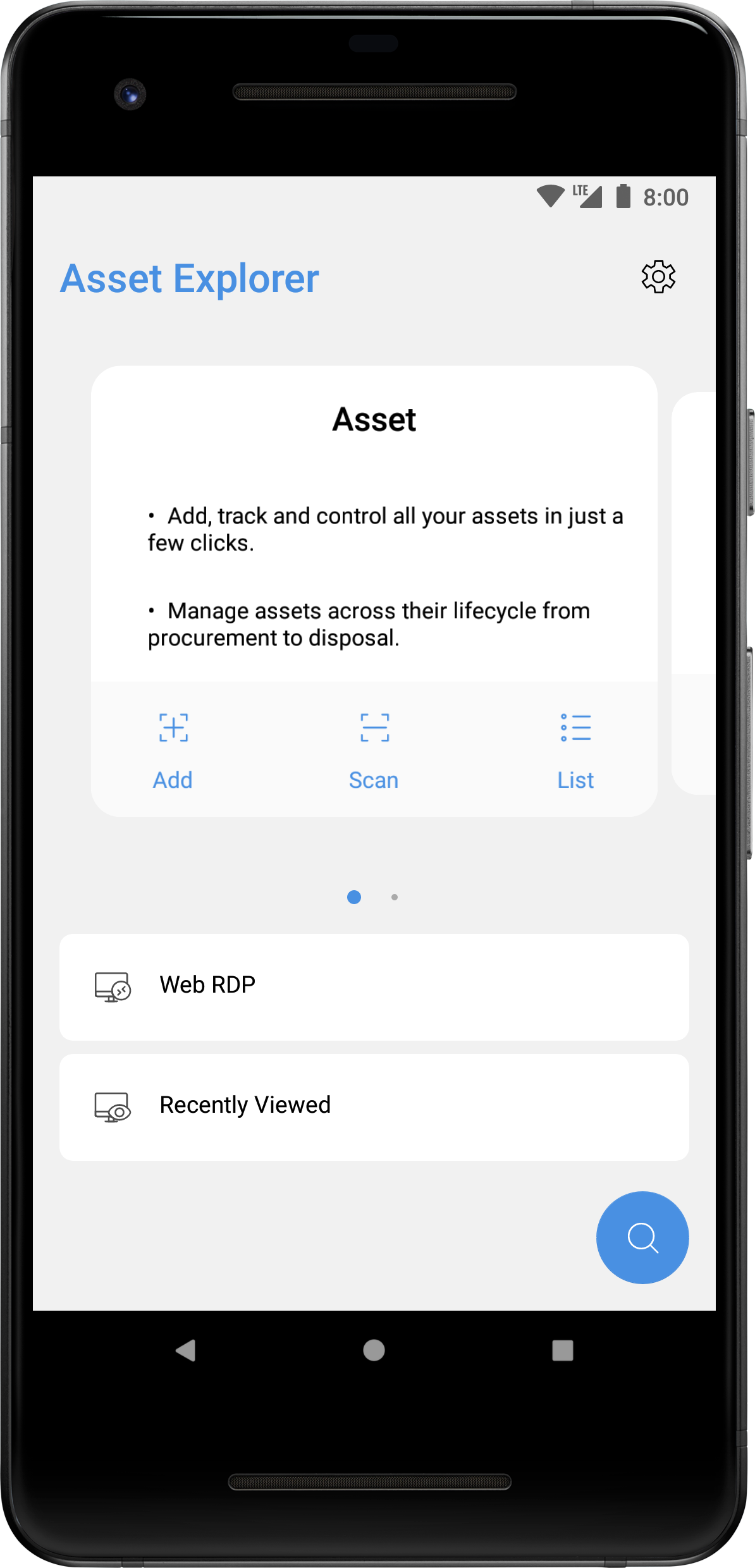A detailed caption of the image would be:

"A close-up photograph of a black smartphone with a detailed display on its screen. The phone shows a fully connected device with icons indicating full Wi-Fi, full battery, and full LTE signal strength in the top right corner. The physical design includes a camera and a speaker at the top and a receiver at the bottom, typical of most smartphones.

On the screen, the application 'Asset Explorer' is prominently displayed on a white background with the title in blue letters. To the right of the title, in the upper corner, there is a gear icon indicating access to the configuration menu. Below the title, within a white box containing black text, it reads "Asset" followed by descriptors such as "add, track, and control all your assets in a few clicks and a minute. Assets across their life cycle from procurement to disposal."

Below this text, there are three blue buttons labeled 'add,' 'scan,' and 'list.' Further down, there is a navigation indicator with a blue dot and a gray dot. Below these indicators are two more white rectangular boxes labeled 'WebRDP', accompanied by a monitor icon, and 'Recently Viewed', which features a monitor with an eye icon next to it.

In the bottom right-hand corner of the screen is a blue circle containing a magnifying glass, symbolizing the search function. The phone's interface also includes the customary back, home, and menu buttons at the bottom of the hardware."

This provides a comprehensive and descriptive caption of the image, highlighting both the physical aspects of the phone and the detailed elements displayed on its screen.